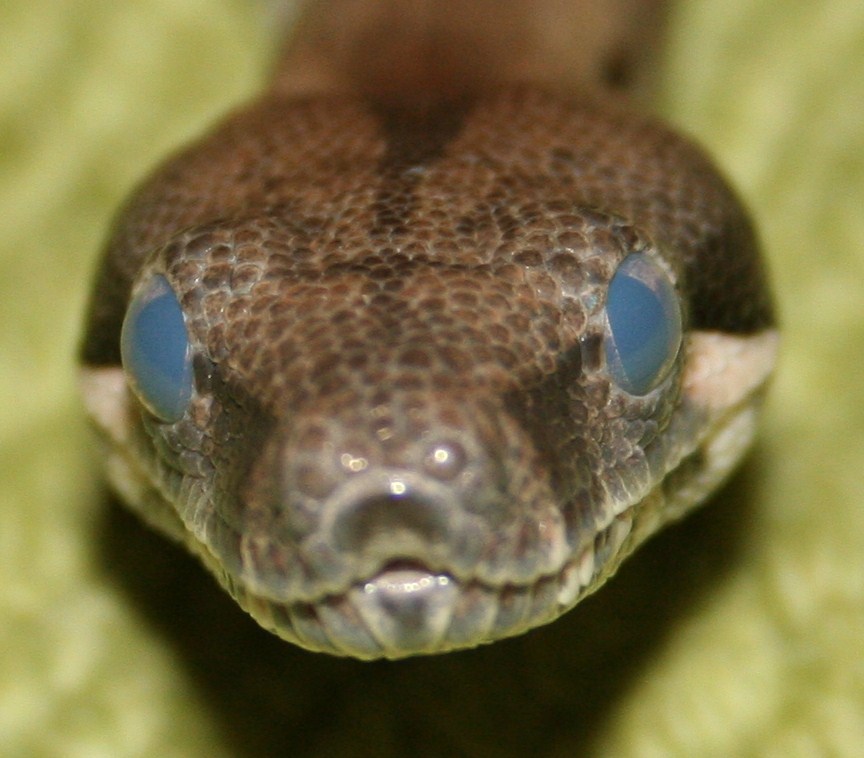The photo captures an extreme close-up of a snake, with its head dominating the frame, occupying about 80% of the image. This snake, possibly a small brown garden snake, is positioned front and center, staring directly at the camera. Its scales bear a pattern of circular, dark and light brown hues, alongside a distinctive black marking on its head that resembles the shape of a lyre or music stand. The snake's eyes are a pallid blue, appearing glossy and perhaps even having a translucent layer akin to an eyelid. Its mouth is closed, and the overall shape of the head is slender yet subtly diamond-like. Although a small portion of the snake's body is visible at the top of the image, it is cropped and out of focus. The background is a blurry but vibrant green, suggesting foliage or leaves, which contrasts sharply with the detailed, textured scales of the snake's head.